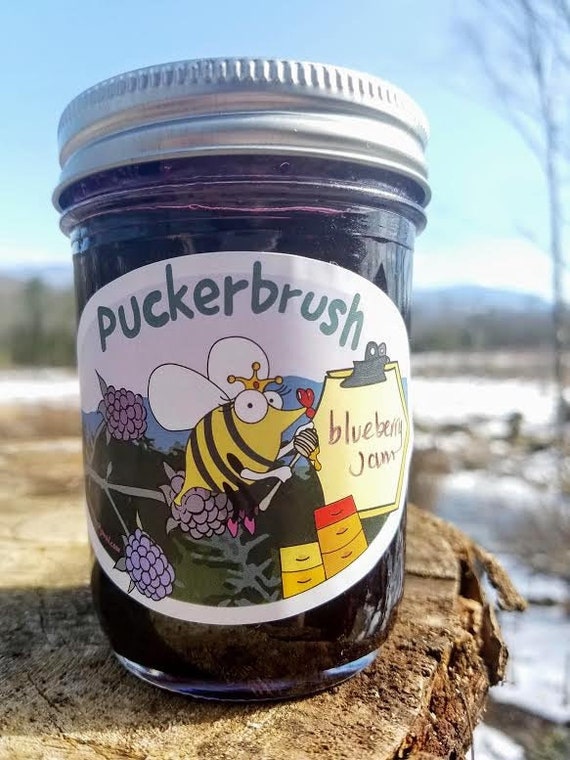This is a close-up outdoor photo of a mason jar filled with purple-colored blueberry jam. The jar has a silver metal lid and sits on a naturally textured wooden surface that resembles the cross-section of a tree trunk. A round, white label on the jar prominently features the words "Pucker Brush" at the top. Below this is a charming, cartoon-style illustration of a yellow and black bumblebee with white wings and a yellow crown. The bee is depicted carrying a honey dipper and a clipboard with "Blueberry Jam" handwritten in black ink. Surrounding the bee illustration are clusters of blueberries. The background of the image is blurred but reveals a glimpse of a distant mountain range under a sunny sky, emphasizing the outdoor setting.